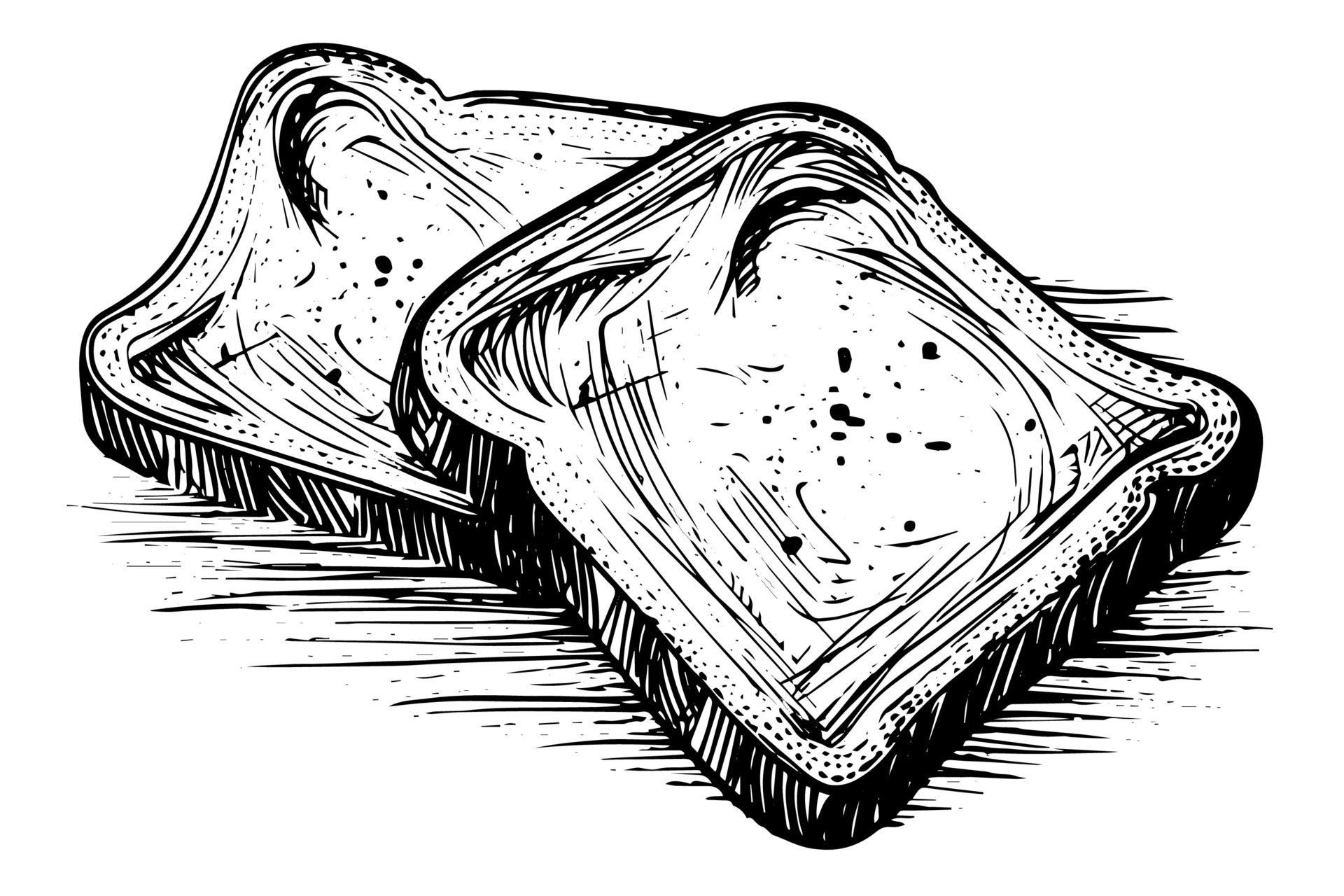The image is a simple, black and white drawing featuring two slices of bread. The slices are sketched in a cartoonish style with rounded edges and are positioned one on top of the other in a slightly jumbled manner. The bread slices have black edges, black lines, and several small, black dots on their surfaces, giving them a textured appearance. The drawing lacks color and detailed elements, making it very plain and subtle. Both slices rest on a surface that is suggested by horizontal shading lines, possibly indicating a tabletop or some other flat surface. The image is minimalistic and doesn't seem to convey much meaning beyond depicting the bread slices. The overall look is very basic and straightforward.